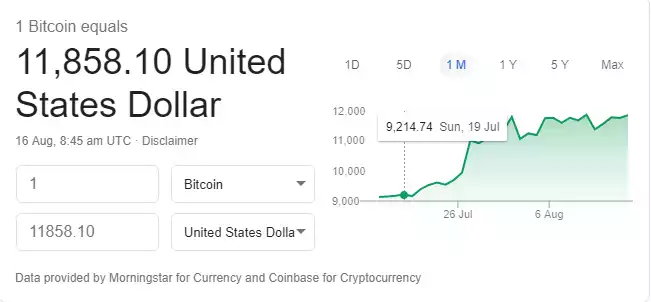A cropped image displaying the current Bitcoin price from a Google search. The background is white. At the top left, in grey letters, it reads "1 Bitcoin equals." Directly below that, in very large black font, the price is shown as "$11,858.10 USD." Underneath, to the left, the time and date are displayed in small grey font, with the word "Disclaimer" to the right. At the bottom left, a text box with the number "1" entered is visible, followed by a drop-down box set to "Bitcoin." Adjacent to it is another text box showing "11,858.10," with a corresponding drop-down box selected to "United States Dollar." At the very bottom left, grey font indicates "Data provided by Morningstar for currency and Coinbase for cryptocurrency." On the top right, there is a line graph, with categories above ranging from "1 day" to "Max", currently set to the center option, "1 month."